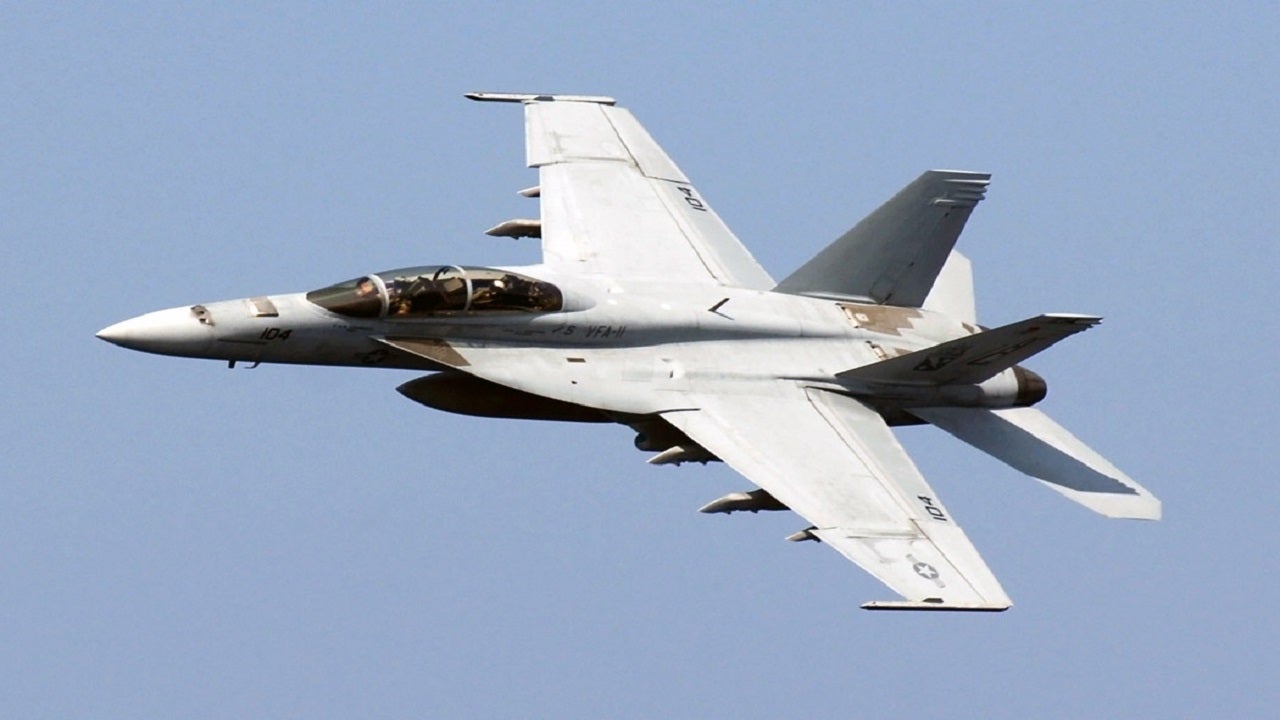In this image, a sleek, silver-gray military fighter jet, adorned with the number 104 on its front left side and both main wings, dominates the clear, light blue sky. The aircraft features a pair of main wings and four tail wings—two positioned further back and two slightly ahead and on top. The jet is likely part of the Air Force, potentially on a mission or reconnaissance, and is equipped with visible missiles under its wings, highlighting its combat-ready status. There are no clouds or other objects in the sky, emphasizing the jet's swift and determined flight as it appears to surge forward through the open air.